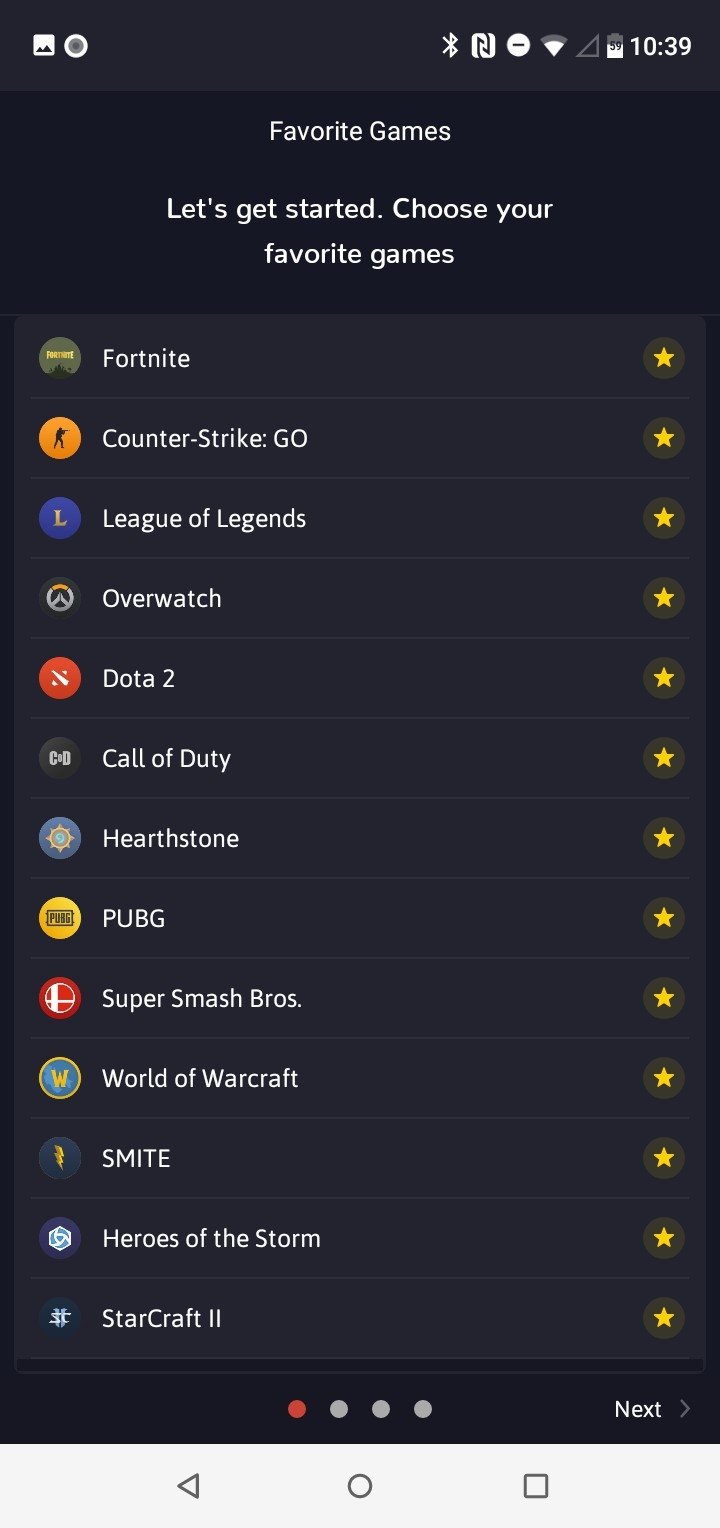This image is a screenshot from a mobile phone interface. The top bar of the screen displays various status symbols, with the battery icon on the right showing a little over half full and a signal strength indicator nearby. The time is clearly visible in the top right corner, reading 10:39. The background of the screenshot is entirely black.

Centered beneath the top bar, in bold white text, are the words "Favorite Games," followed by an invitation to "Let's get started, choose your favorite games." Below this text is a vertical list of popular game titles, each accompanied by its respective logo and a star icon to the right, which is either yellow or orange in color. The games listed include:

- Fortnite
- Counter-Strike: GO
- League of Legends
- Overwatch
- Dota 2
- Call of Duty
- Hearthstone
- PUBG
- Super Smash Bros.
- World of Warcraft
- Smite
- Heroes of the Storm
- StarCraft II

Each game logo is distinctive, such as Counter-Strike's emblem featuring a person in an orange circle.

At the bottom of the screen, there are four circles indicating pagination, with the leftmost circle highlighted in an orangish red, suggesting this is the first page. To the right, a "Next" button indicates the availability of additional pages of games. 

The bottom-most section of the screen includes a back arrow, a home button, and a tab button, allowing the user to navigate to different tabs. This detailed layout and information make it clear that the user is on a selection page for their favorite games within an application.